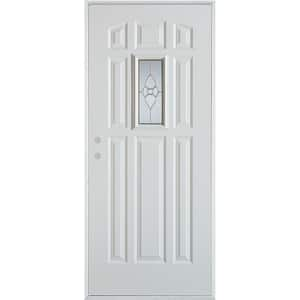This image depicts a standard front door, likely photographed from the interior side, showcasing its distinct features in detail. The door is white with three columns of rectangular embossments arranged in three rows, each progressively larger from top to bottom. The bottom row features the longest embossments, around three feet in length. The middle row includes a slender, rectangular stained glass panel located centrally, adorned with a semi-circular design and two leaf-like patterns. The top row comprises smaller, more squared-off embossments. The door lacks a doorknob, displaying two holes where a knob and lock would typically be positioned on the left side. The narrow frosted glass panel, positioned in the upper half of the door, adds an elegant touch with its intricate floral design, enhancing the overall aesthetic of the entryway.